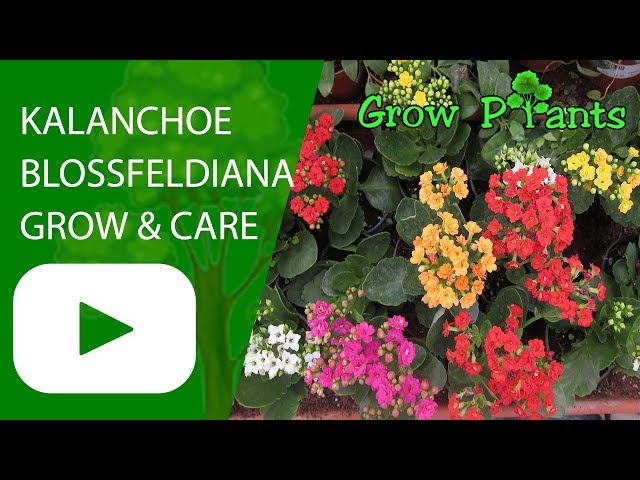The image is a vibrant and inviting YouTube video thumbnail regarding plant care. Split into two distinctive halves, the left side features a bright, grass-green translucent area with the YouTube Play logo and white text that reads "Kalanchoe Blossfeldiana Grow and Care." Above the arrow in white letters is the brand name. The right side showcases a visually appealing close-up of a potted plant with lush dark green leaves and an array of colorful flowers, including shades of light orange, red, bright pink, white, yellow, and purple. Notably, on the top right corner, the words "Grow Plants" appear, with "Grow" in neon green text and "Plants" incorporating a cartoon tree in place of the letter "L." The overall presentation is colorful and engaging, clearly aimed at providing information on how to care for Kalanchoe Blossfeldiana plants.